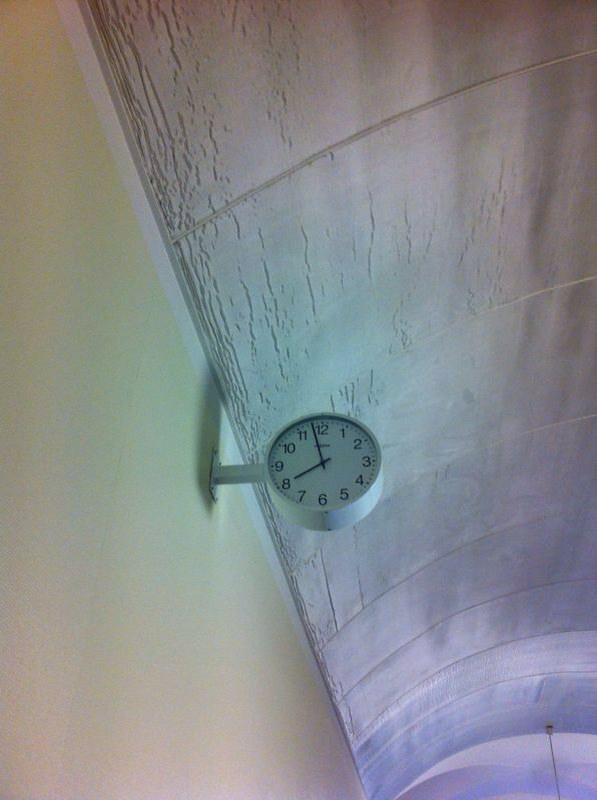This detailed photograph captures a scene where a vaulted, rounded ceiling and a section of a wall meet in a hallway-like area. The ceiling is predominantly white with visible cracks and transitions to a variably colored section featuring hues of pink, purple, and bluish tones, especially evident in the bottom right corner of the image. Hanging from the ceiling, a chain or rope extends downwards, possibly connected to a light fixture.

The wall, which is a yellowish-tan or light creamy color, features a prominently mounted white clock. This clock is affixed to the wall using a small metal bracket or a silver cylindrical post, giving it a slight protrusion. The clock itself has a clean white face, black traditional numbers ranging from 1 to 12, and black hour and minute hands. The time displayed is just before 8 o'clock, with the small hand on the 8 and the large hand approaching 12. The overall impression is reminiscent of a utilitarian space, similar to what one might encounter in public areas such as airports.